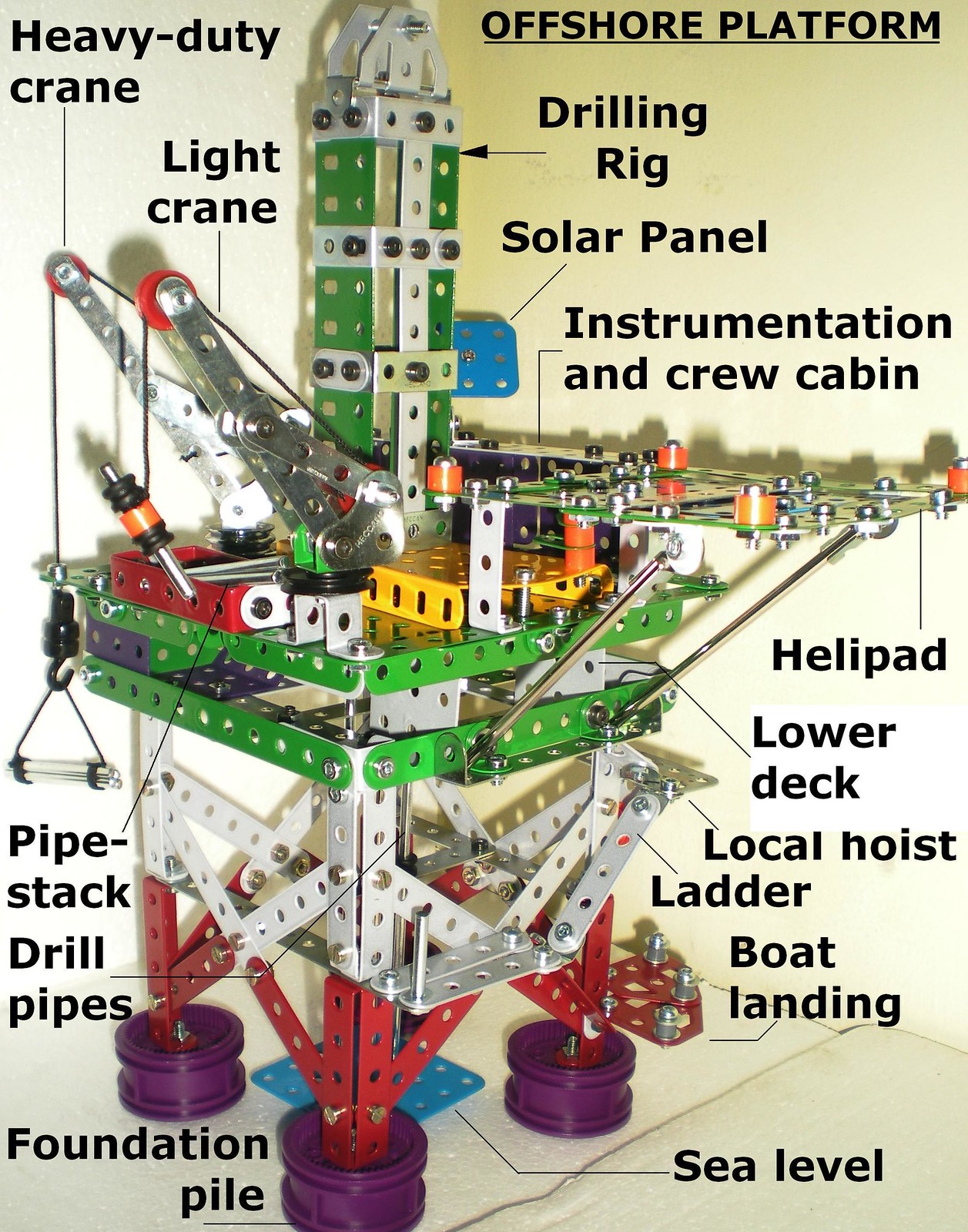This is a vertical rectangular poster showcasing a detailed illustration of a toy offshore oil platform. The title "Offshore Platform" is prominently displayed in the upper right corner in black, underlined text. The central part of the image features a meticulously assembled replica of the platform, composed of various metal scraps and straps bolted together. The base of the platform consists of cylindrical purple objects and strong, red and silver steel columns that support the entire structure.

The main platform is green and houses a big silver heavy-duty crane and a light crane on the left, as well as a green tower. Additional elements include the drilling rig, solar panel, helipad, and a clearly marked sea level. Each component of the model is carefully labeled with black arrows pointing to their respective parts. Key labels include the heavy-duty crane, light crane, drilling rig, solar panel, instrumentation and crew cabin, pipe stack, drill pipes, foundation pile, helipad, lower deck, local hoist ladder, boat landing, and sea level. This detailed labeling makes it an educational and engaging toy for children.